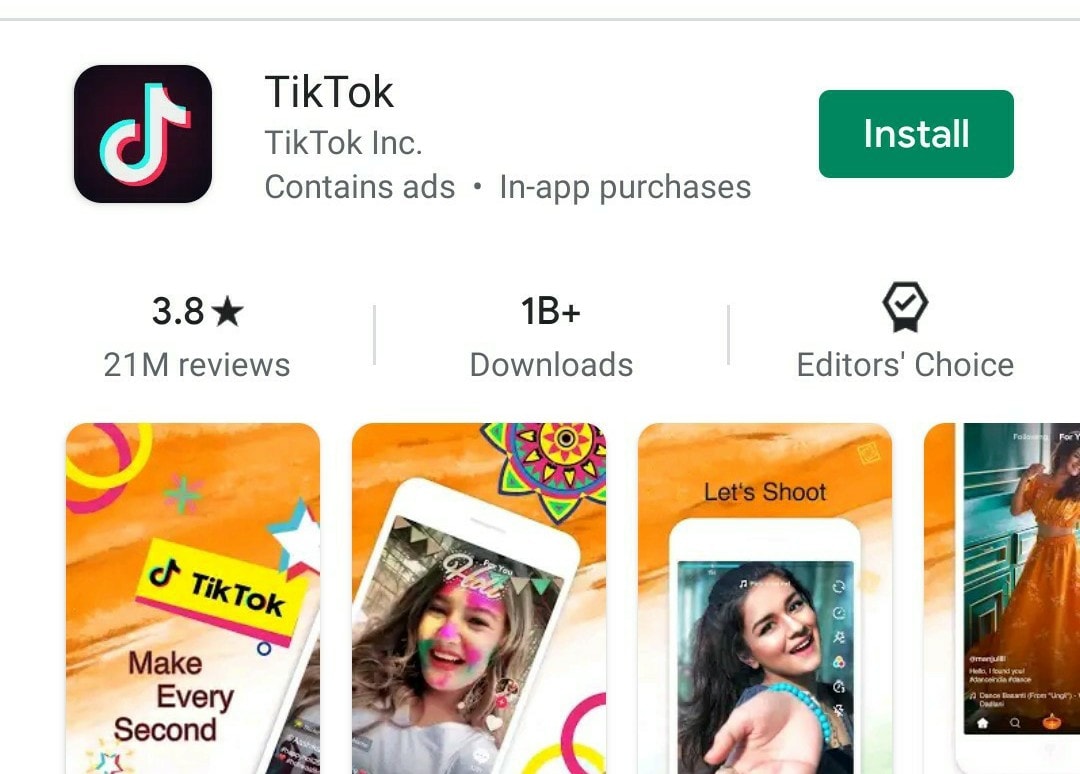Caption: 

A detailed screenshot of the TikTok app's listing on the Google Play Store. At the top left, the recognizable TikTok logo is prominently displayed. To the right of the logo, the app's name "TikTok" is clearly visible. Underneath, it states the developer as "TikTok Inc." Following this, there's a line indicating the app contains ads, represented by a small gray circle. Additionally, it mentions the availability of in-app purchases. On the right side, a prominent green "Install" button is shown in white text, inviting users to download the app. Towards the bottom left, the app's rating is displayed as 3.8 stars, and it boasts over 1 billion downloads. The listing also highlights that TikTok is an "Editor's Choice" app.